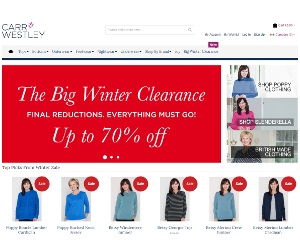The image appears to showcase a shopping website named "Car Wesley." Positioned at the top left, the website name is prominently displayed. In the top middle section, a search bar is situated, flanked on the far right by a magnifying glass icon to facilitate searches.

Centrally located on the page is a large, attention-grabbing rectangular banner with a vibrant red background. The banner prominently features the text "The Big Winter Clearance" in bold lettering. Beneath this, it states "Final Reductions, Everything Must Go," highlighting significant markdowns. Below this, an enticing "Up to 70% off" offer is displayed. Further down the banner, two noticeable circles—one large and one small—are present, potentially indicating featured items or important announcements.

Directly below the banner are images of six women showcasing different pieces of clothing. On the bottom left, a woman with long black hair dons a blue long-sleeved shirt. Adjacent to her on the right is a white woman dressed in a very bright long-sleeved blue shirt. Following her, the same woman from the first image appears again, this time in a greenish-blue sweatshirt. Next, another woman is seen wearing a black sweatshirt. The fifth image features the same greenish-blue sweatshirt as previously shown. In the last image on the bottom right, a woman is wearing a white jacket over a white shirt, completing the diverse array of clothing items displayed.